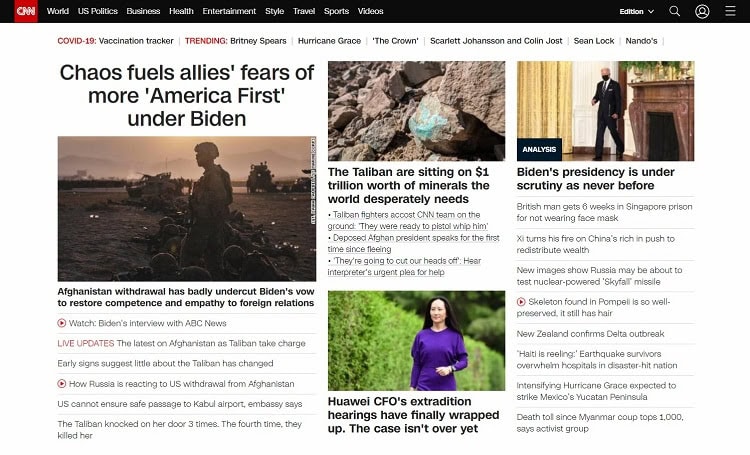Screenshot from the CNN website:

The screenshot prominently features the CNN logo in the upper left-hand corner, which is white text on a red square inset on a large black header bar. The bar contains their menu options: World, U.S. Politics, Business, Health, Entertainment, Style, Travel, Sports, Videos—all in white text. On the right side of the header, there is an additional section with a drop-down option, a magnifying glass icon, a profile image, and a hamburger menu.

Beneath the header, several headlines are displayed, separated by vertical gray bars. In red text, it reads "COVID-19," followed by "Vaccination Tracker" in black. To the right, in red bold caps, "TRENDING," and subsequent headlines include "Britney Spears" in black, followed by "GOP" in red, "Hurricane Grace," "The Crown" in quotes, "Scarlett Johansson and Colin Jost," and "Sean Locke" followed by "Nando's."

The content is displayed in three columns—the left one being slightly wider than the other two:

1. **Left Column:**
   - Headline: "Chaos Fear Allies Fears of More, America First," with "America First" in bold and in quotes.
   - Below the headline, an image of a soldier standing with tanks and other armored vehicles in the background, with men laying on the ground in sand.
   - Caption: "Afghanistan withdrawal has badly undercut Biden's vow to restore competence and empathy to foreign relations."
   - A section with live updates and options is presented below.

2. **Center Column:**
   - Headline: "The Taliban are sitting on $1 trillion worth of minerals the world desperately needs."
   - Image: Rocks with some blue coloring.
   - Below are additional links.
   
3. **Right Column:**
   - Image of an Asian woman in a purple shirt with long hair, walking.
   - Headline: "Huawei's CFO's extradition hearings have finally wrapped up, the case isn't over yet."
   - Image of Biden wearing a COVID mask with an "Analysis" button overlay.
   - Caption: "Biden's presidency is under scrutiny as never before."
   - Additional options presented below in text.

The screenshot provides a detailed overview of the main stories and sections on the CNN website at the time, focusing on current events, political news, and major global headlines.